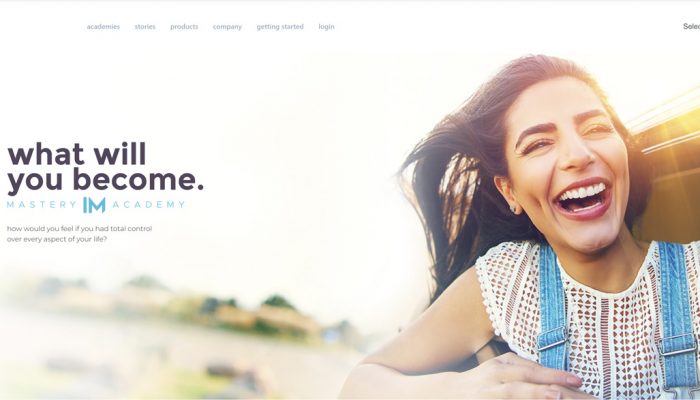**Screenshot of Mastery Academy Website Homepage**

The homepage of the Mastery Academy website features a vibrant and engaging layout. At the top, a navigation bar displays menu options: *Academy, Stories, Products, Company, Getting Started,* and *Log In*. 

The main focus of the image is a spirited woman possibly sticking her head out of a moving car, with the wind playfully tousling her hair. She is bathed in the warm, golden light of the setting sun, which reflects in her joyous eyes. She is dressed in casual, farmer-inspired clothing, including overalls, and her face is lit up with an exuberant, wide smile.

To the left of the woman is a blurred background that hints at a neighborhood setting, adding depth to the scene. 

A motivational message overlays the image: "What will you become Mastery Academy?" with a blue "M" logo nestled between the words "Mastery Academy." Below, the text poses an intriguing question: "How would you feel if you had total control over every aspect of your life?"

In the top right-hand corner, partially cut-off text appears, possibly reading "Select". 

Overall, the design invites visitors into an inspiring journey towards personal empowerment and mastery.